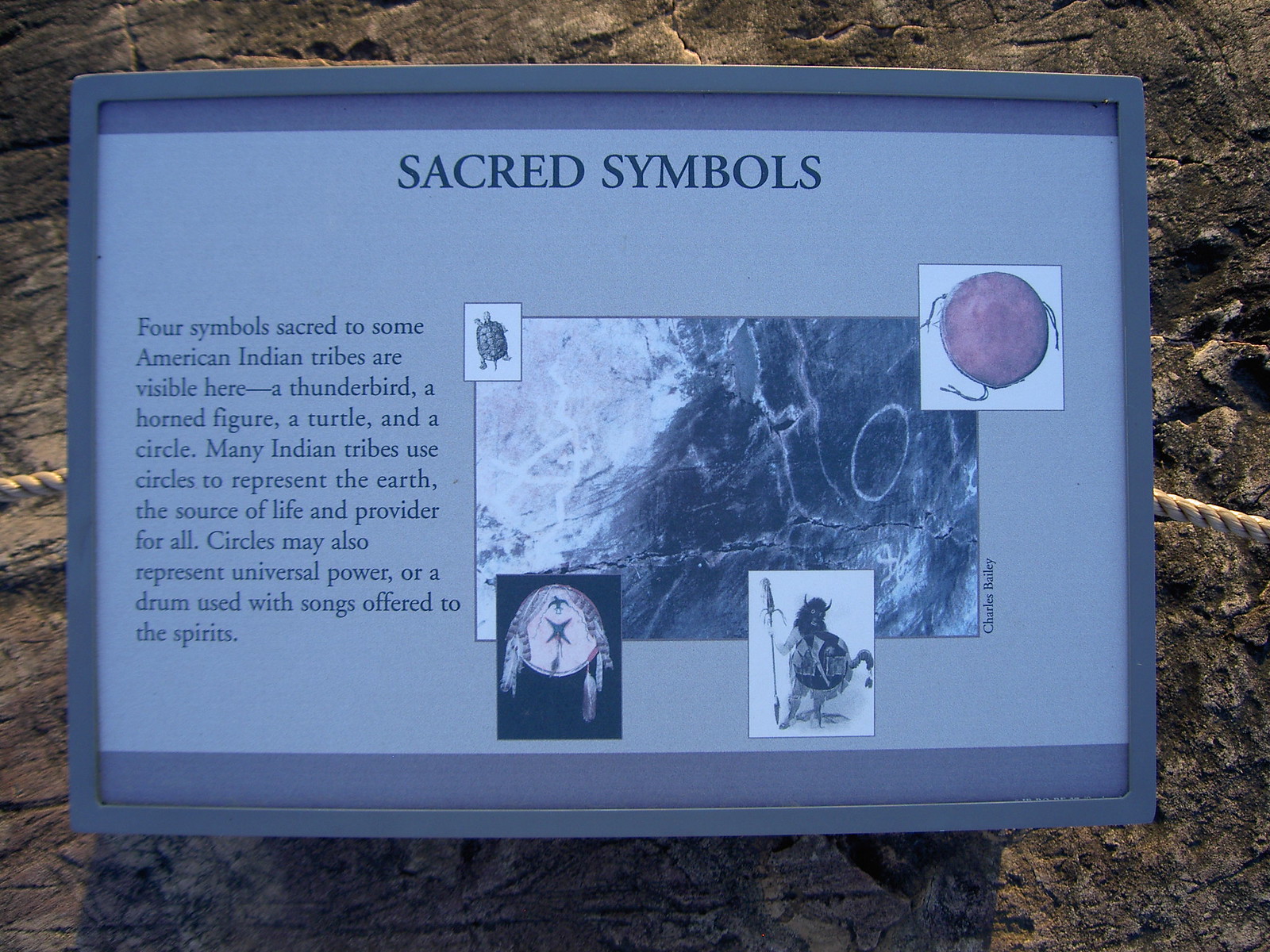This image captures a sign at a museum, mounted against a textured dark gray rock surface with flecks of gold. Framed in a gray metal or plastic border, the sign has a light gray background with darker gray text and accents. It is held in place by light brown ropes on either side. At the top of the sign, bold black capital letters read "SACRED SYMBOLS." Beneath the title, the left side features a paragraph explaining that four symbols sacred to some American Indian tribes are depicted: a thunderbird, a horned figure, a turtle, and a circle. The text further explains that circles are often used by many Indian tribes to represent the earth, symbolizing the universal source of life and power, or a drum used in spiritual songs. To the right of the text, there is a large central image showing rock wall drawings of various objects, accompanied by four smaller images below it, which include depictions of a turtle, a red circle, a horned figure, and what appears to be a drum or tambourine.